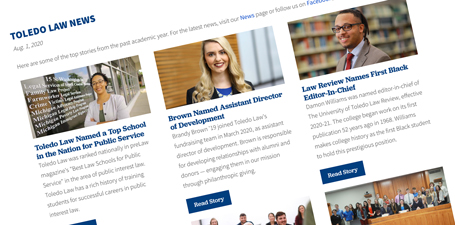This image displays a section of a news website with highlighted articles from "Toledo Law News." At the top, "Toledo Law News" is prominently featured in blue text, followed by the publication date, August 2, 2020, alongside a short, less legible sentence in gray with two notable blue words. Below this header, three main articles are showcased.

1. The first article is titled "Toledo Law Named a Top School in the Nation for Public Service."
2. To the right of it, the next article reads "Brown Named Assistant Director for Development."
3. Further right, the final article is "Law Review Names First Black Editor-in-Chief."

All titles are presented in blue text, followed by a brief descriptive paragraph in gray. Under each paragraph is a blue rectangular button bearing the text "Read Story" in white.

The image includes headshots of three individuals, one for each article. The layout reveals:
- The bottom left article is partially visible, showing a small blue sliver.
- The middle article is cut off, showing about half of its top portion.
- The rightmost article displays roughly 60% of its top portion.

A clean white background frames the entire layout, providing a clear and organized presentation of the news articles.